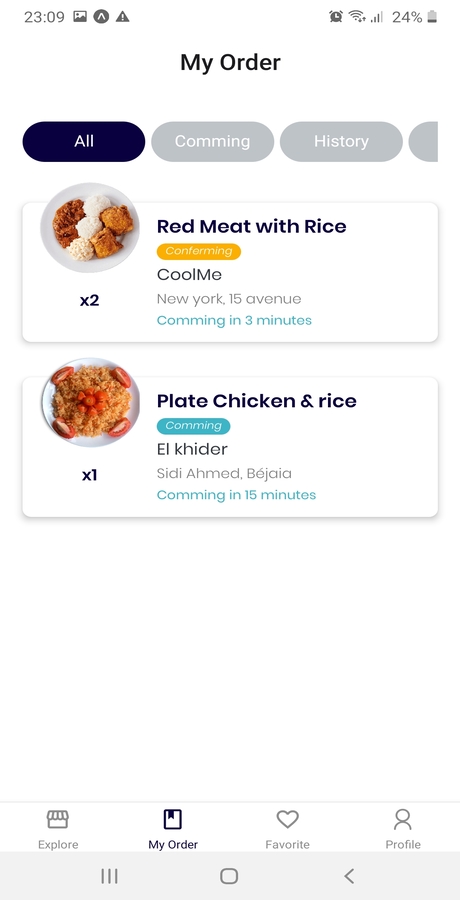**Detailed Caption:**

The image appears to be a screenshot from a cell phone taken at 23:09. The top of the screen shows several status icons, including an alarm clock symbol, Wi-Fi signal, cell signal, and a 24% battery indicator. The app displayed is likely a food delivery service, given the content.

The primary heading on the screen reads "My Order," and there are tabs titled "All," "Coming," and "History." The "All" tab is highlighted in blue with white text, while the other tabs feature white text on a gray background.

There are two active orders displayed on this screen:

1. The first order is listed at the top with a red meat and rice dish. This entry has a blue background and white text, including a yellow oblong button labeled "Confirming." The order is from "Cool Me, New York, 15 Avenue," and it's estimated to arrive in three minutes. The entry notes there are two servings of this dish, as shown with a small icon of a plate of food next to the details.

2. The second order below lists chicken and rice, with the origin "Elk Kinder, K H I N D E R, Sid Ahmad Ben Jad, Sidi Ahmad, A H M E D Benji B E J A I A." This order is expected to arrive in 15 minutes with one serving, and there's also an icon depicting a plate of food.

At the bottom, the app's navigation bar includes options for "Explore," "My Order," "Favorites" (indicated by a heart icon), and "Profile." Below this, there is the phone's navigation bar with three vertical lines, a circle (probably the home button), and a backward arrow (likely the back button).